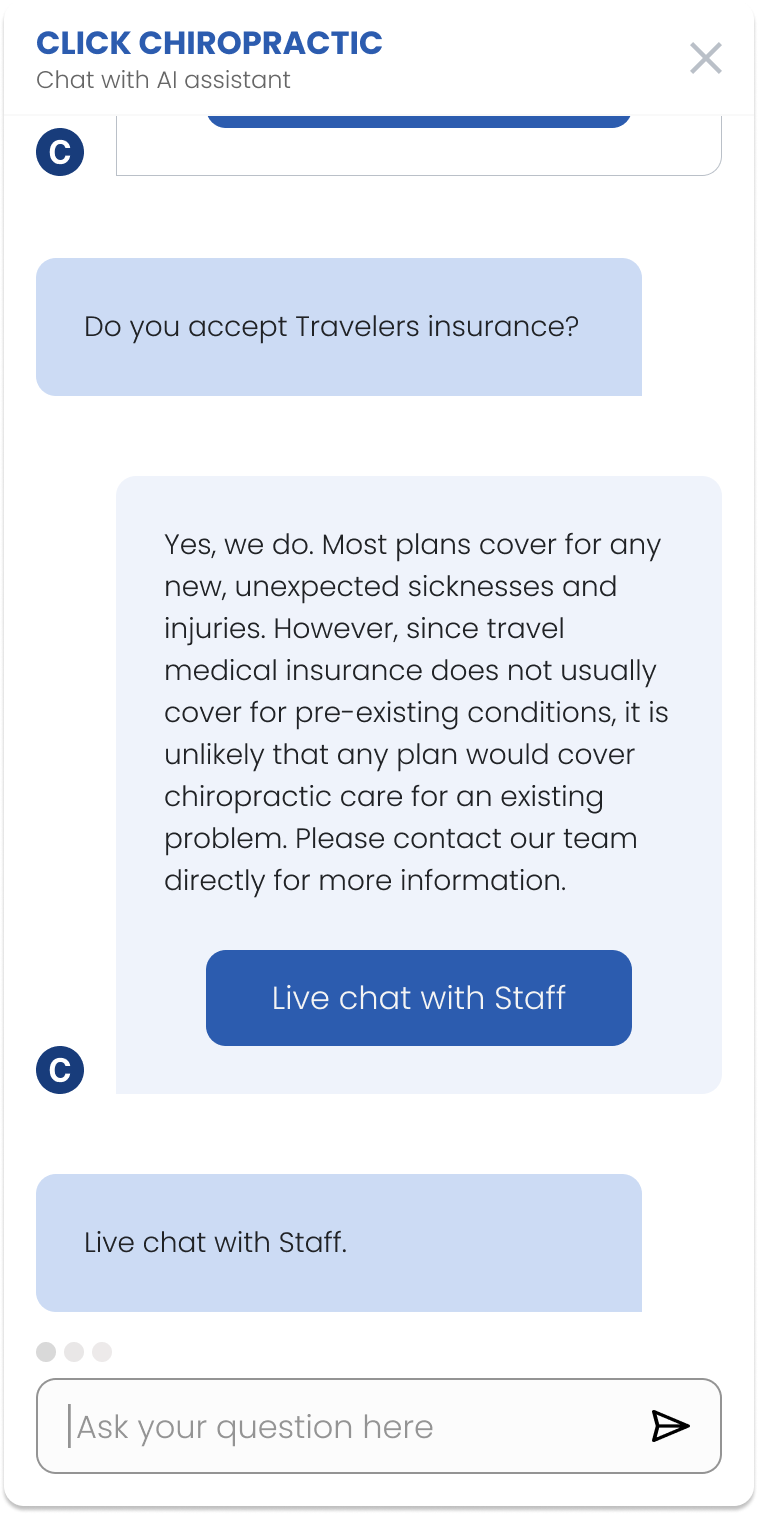The image depicts a user interface of a chiropractic service named "Click Chiropractic" featuring a chat with an AI assistant. In the upper left-hand corner, the title "Click Chiropractic" is prominently displayed next to an option labeled "Chat with AI Assistant." The main section of the image shows a conversation between a user and the AI assistant. Although the top part of the conversation is partially cut off, the visible segment reveals a dialogue box where the user has asked, "Do you accept travelers insurance?" 

This user question appears in a bluish speech bubble, characterized by a curved shape on three sides and a pointed edge on one side, mimicking the aesthetics of a traditional speech bubble. The AI assistant's response is displayed below, stating: "Yes, we do. Most plans cover for any new unexpected sicknesses and injuries. However, since travel medical insurance does not usually cover pre-existing conditions, it is unlikely that any plan would cover chiropractic care for an existing problem. Please contact our team directly for more information."

At the bottom of the screen, a prominent clickable box invites users for a "Live chat with staff," further facilitating direct interaction.